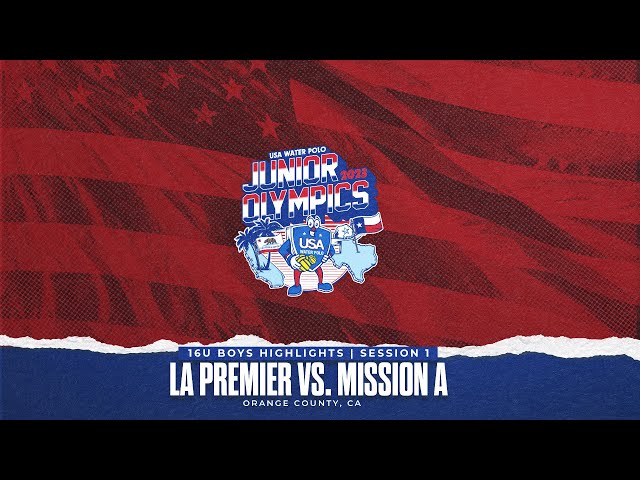The image appears to be a screenshot from a video advertisement promoting the USA Water Polo Junior Olympics 2023 event. The layout features black bars at the top and bottom, giving it a cinematic feel. Dominating the center is a blurred, maroon-tinted United States flag, stylized and monochromatic. Layered over this backdrop is a prominent blue shield logo with a cartoonish mascot that has arms and legs, emblazoned with "USA" in white. Above the mascot, bold text reads "USA Water Polo Junior Olympics 2023." Flanking the mascot, there's an illustrated Texas on the right with a Texas flag and palm trees on the left representing Florida. Beneath this is a torn-paper effect in blue, containing the text "16U Boys Highlights Session 1" in blue lettering. Below that, even larger white font declares "LA Premier versus Mission A," with "Orange County, CA" in smaller capital letters, indicating the event location.